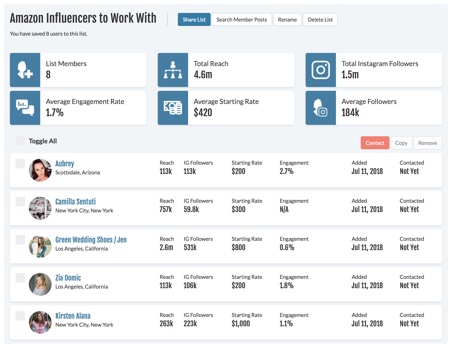The image depicts a user interface for managing Amazon influencers, displaying various details about the influencers that a user has liked. At the top, a gray bar contains the title "Amazon Influencers," accompanied by options to share the list and search for a member. Below this, there's a hard-to-read instruction in small print, and additional options to describe and list members. Key metrics such as "Total Reach," "Total Instagram Followers," "Average Engagement Rate," "Average Starting Rate," and "Average Followers" are prominently displayed with blue icons on their left.

Towards the bottom, the interface lists individual influencers. Each influencer's section starts with a small gray box next to their name, followed by their profile picture. Their respective statistics are displayed in light green across the width of the white box that contains all their details. Additionally, there is a "Contact Them" button in orange, allowing users to reach out to the influencers. The list of influencers is presented in an organized format, making it easy to toggle between different entries.